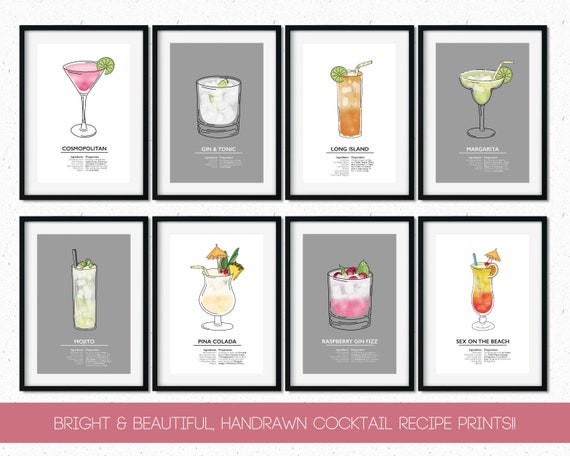This set of images showcases various hand-drawn cocktail recipe prints, each neatly framed in black borders. At the center of each frame, vibrant and colorful illustrations of classic cocktails are meticulously detailed, including a Margarita, Long Island Iced Tea, Gin and Tonic, Cosmopolitan, Piña Colada, and Sex on the Beach. Beneath each visually striking drink, there are descriptive labels and ingredient lists, guiding the viewer on how to recreate these drinks. The frames are labeled at the bottom with the phrase: "Bright and Beautiful Hand-Drawn Cocktail Recipe Prints," emphasizing the artistic and informative nature of these pieces. The vibrant hues of the drinks stand out against the black frames, capturing the essence and allure of each cocktail.